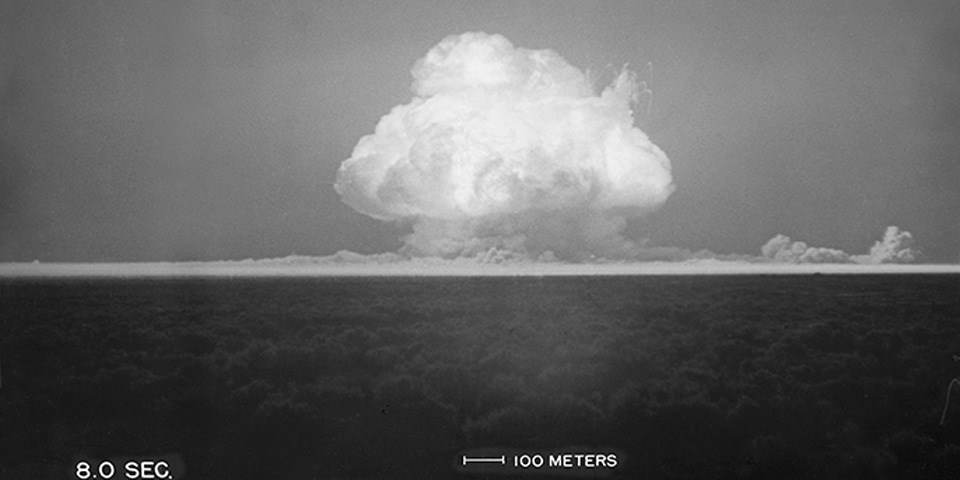A stark black and white photograph captures the moment an atomic bomb explodes, reminiscent of the Hiroshima blast. Central to the image is a colossal mushroom cloud, rising dramatically from the ground and radiating intense brightness at its core. The explosion encompasses a vast area, potentially spanning several hundred meters in diameter. The sky above is a flat gray, contrasting with the white-hot center of the detonation. Surrounding the explosion, clouds and a percussion wave are visible, pushing outward from the epicenter. The foreground appears to be a desolate desert landscape, adorned sparsely with shrubbery. At the bottom of the photograph, text indicates "8.0 seconds" and a measurement bar of "100 meters," providing scale to the enormity of the blast. No human figures or annotations are present, lending a haunting, isolated atmosphere to the scene.